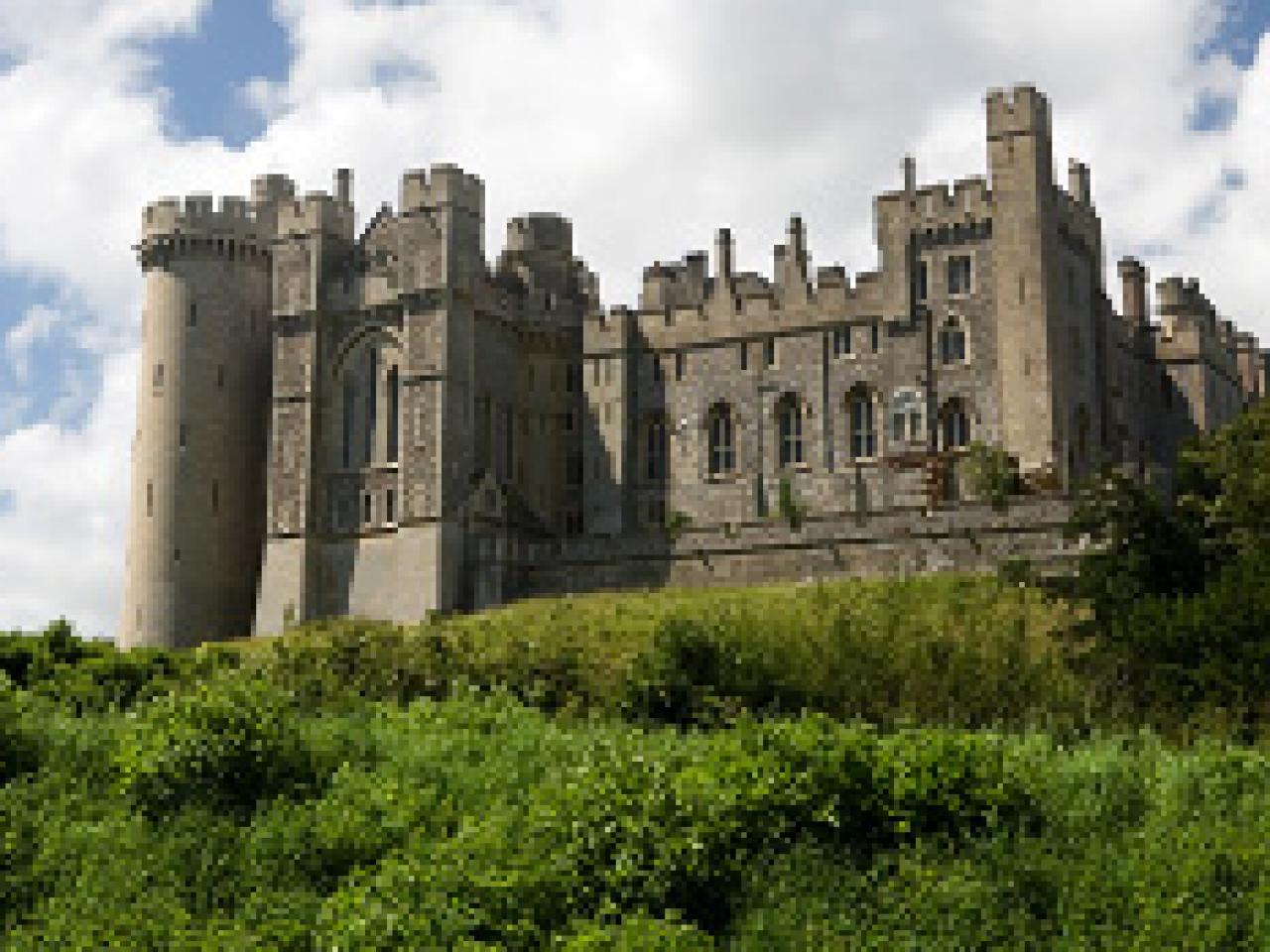The image captures a grand, medieval stone castle set high on a hill, viewed from the front. The structure, predominantly gray in color, features an array of Gothic and square windows, multiple parapets, and several chimneys, suggesting centuries of renovations and additions. Dominating the left side is a round turret, further enhancing the castle’s formidable appearance. The foreground is lush with overgrown green vegetation, rolling hills, and dense foliage, adding to the scenic beauty of the setting. Above, the sky is partly cloudy with large, fluffy white clouds and patches of blue, indicating a bright, sunny day. Despite the image being highly pixelated, possibly due to a poor save or digital editing, the castle’s detailed architecture and the vibrant landscape are distinctly recognizable, giving it a nostalgic, almost video game-like quality.